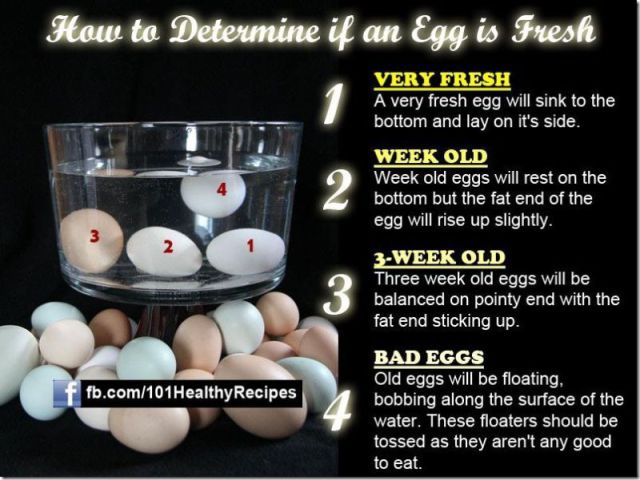**Descriptive Caption:**

A detailed infographic designed for social media, specifically a Facebook graphic, is set against a solid black background. At the top, the graphic features a luminous, cursive white font with the text "How to Determine If an Egg is Fresh." 

To the left side of the image, a tall, elegant, footed glass bowl is prominently displayed. The bowl, elevated by a sturdy stem, contains four eggs, each numbered for clarity. The numbers indicate their position and floating status within the bowl:

- **Egg 1**: Lying on the bottom of the bowl to the right (labeled as very fresh).
- **Egg 2**: Resting at the center of the bowl.
- **Egg 3**: Positioned on the left side of the bowl.
- **Egg 4**: Floating near the surface of the water.

Encircling the base of the glass bowl is a collection of various white and brown eggs. On the right side of the image, the numbers 1 through 4 are listed vertically, each accompanied by a description of the egg’s freshness denoted by its position in the bowl:

- **1 - Very Fresh**: A very fresh egg will sink to the bottom and lay on its side.
- **2, 3, and 4**: Further descriptions detail the process of identifying the age of an egg by its buoyancy.

At the bottom left corner of the graphic, a black rectangular banner provides additional information, showcasing the Facebook page: fb.com/101healthyrecipes.